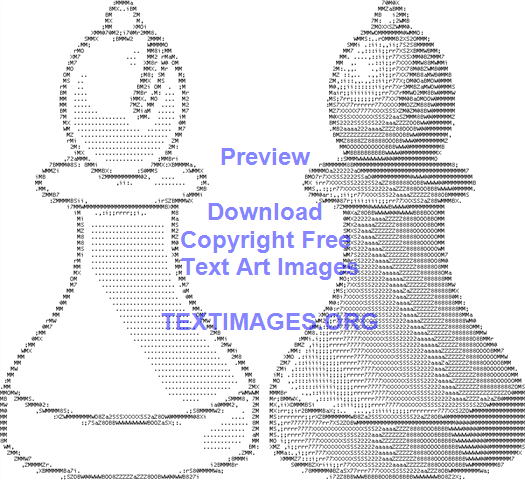The image features two artistically sketched chess pieces, resembling bishops, created using ASCII art, which involves composing images from letters and characters such as Z, X, S, and A, repeated over and over again. The chess pieces are positioned side by side, with the lighter, less shaded one on the left, and the darker, more shaded one on the right. Blue text overlays the center of the image, reading: "Preview. Download copyright-free text art images," and at the bottom, "textimages.org." The advertisement invites viewers to explore and download these impressive text-based images from the provided URL.